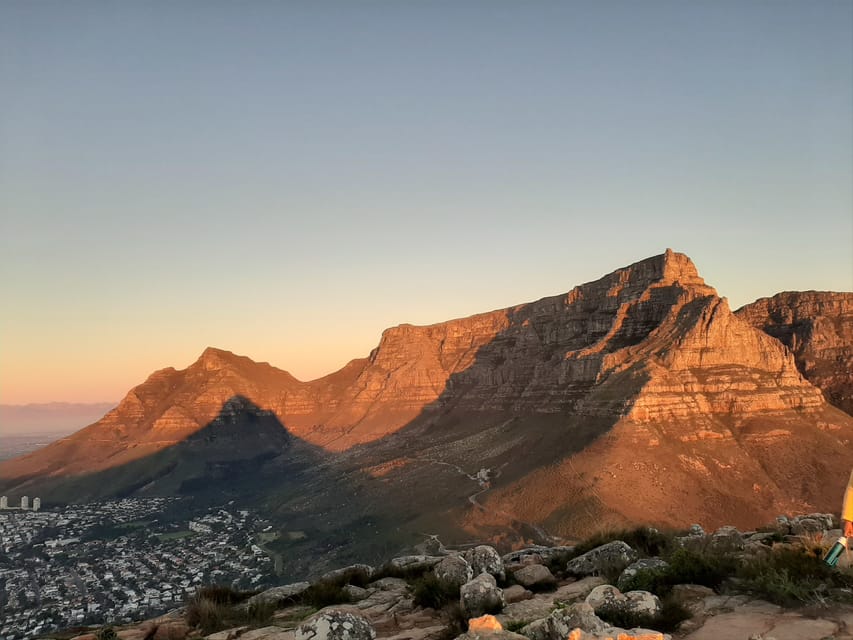The photograph captures a stunning, rocky desert scene dominated by a massive beige mountain reminiscent of the Grand Canyon, with hints of orange clay and textured layers of stone that illustrate the earth’s natural history. The shot, taken outdoors during sunset, bathes the mountain in a golden light. At the base of this colossal formation, a sprawling city with clusters of white buildings is visible, providing a striking contrast against the rugged landscape. The foreground is a rocky area with varied colored stones—white, gray, and more—alongside sparse vegetation and some grass. On the right side, a solitary figure walks, partially obscured but identifiable by a yellow shirt and green boots, holding a blue water jug. The sky above transitions beautifully from a sunset yellow to green, and finally to a deep blue, setting a majestic backdrop for the scenery. The overall atmosphere conveys both the beauty and the challenging terrain of this expansive and picturesque desert valley.